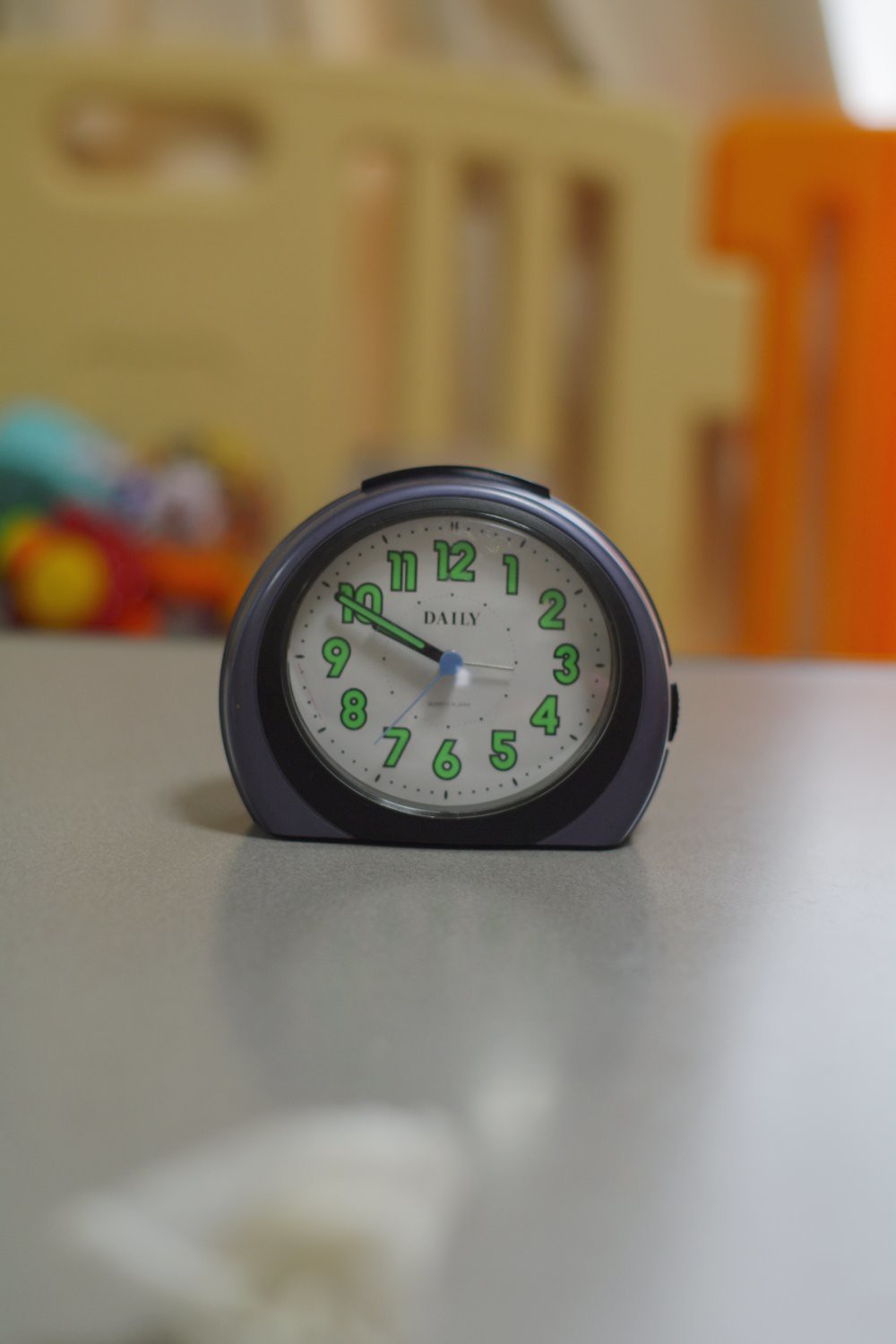The image depicts a small, analog desk clock with a predominantly gray, rounded housing that's flat at the bottom. The clock face is white and features bright neon green Arabic numerals that likely glow in the dark. Both the minute and hour hands are black with neon green stripes down the middle, making them also glow in the dark. The second hand is light blue. At the time captured in the image, the clock shows 10:10. The clock has two black buttons: a long one on the top and a smaller one on the right side, indicating it could be an alarm clock. The clock is resting on a white table in a background that's out of focus, revealing a children's plastic playpen and some blurred, colorful toys, including what seem to be two plastic chairs, one tan, the other orange.